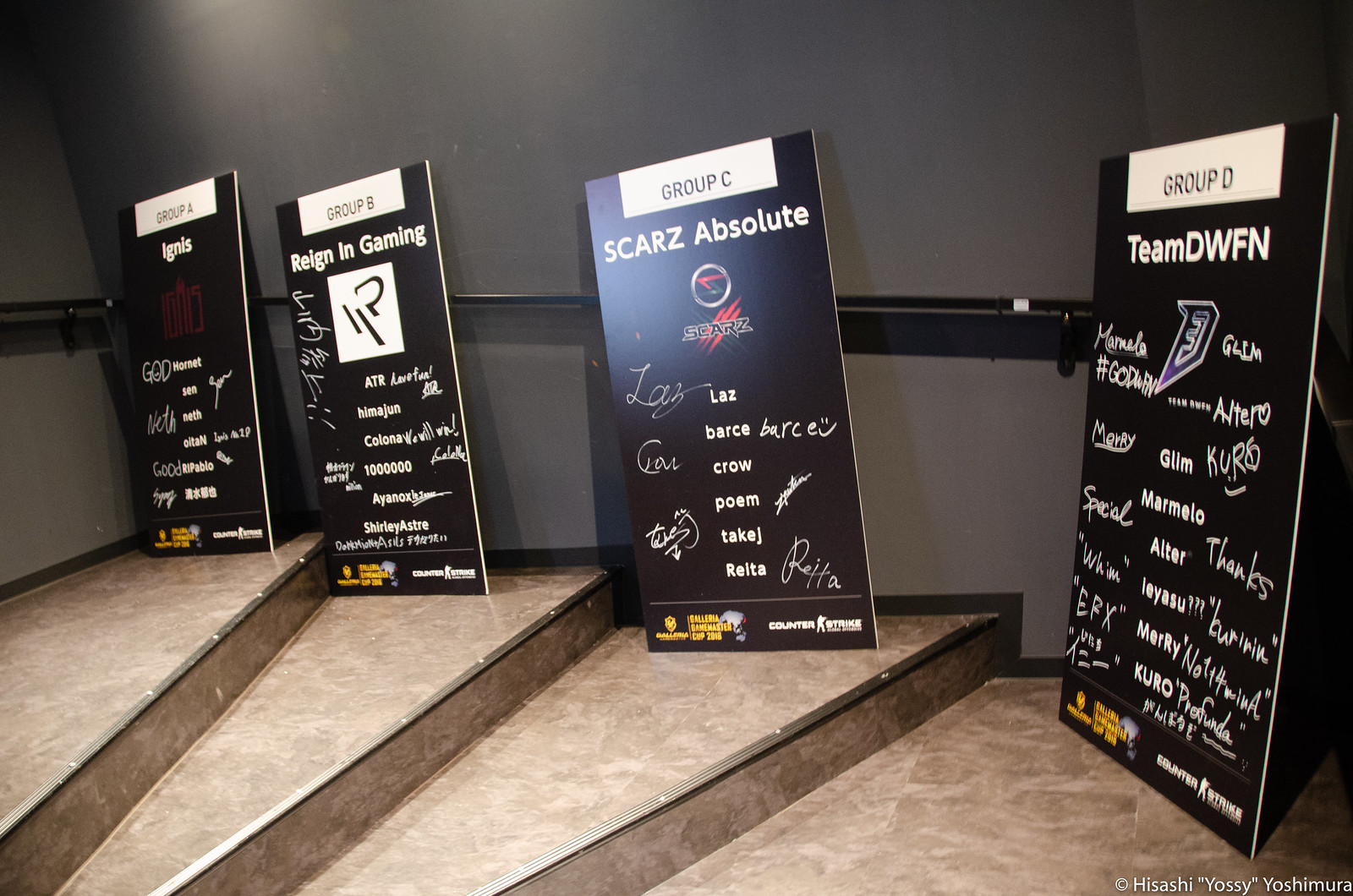This image captures an interior scene with a set of light brown, marble-textured stairs bordered by metallic trim, leading up four levels. Leaning against the gray wall with a black railing that runs horizontally through the middle, there are four vertically oriented rectangular posters, each corresponding to one stair level. The posters are predominantly black with white text and splashes of red, purple, and yellow. 

From left to right, the posters detail the lineups of different gaming groups, likely from a tournament setting:

- **Group A**: Ignis features team members such as God Hornet, Sen Sen, Ness Ness, Otan, Iowas, Good, RIP, and Abloh.
- **Group B**: Reignin Gaming includes ATR, Have Fun, Imogen, Kelowna, A Million, Numbersa, Ionox, Surely, and Astra, with a note mentioning Counter-Strike.
- **Group C**: SCARS Absolute lists members like SCARS Laz, Bars, Crow, Poem, Take J, and Rieta.
- **Group D**: Team DWFN comprises Manila, Godwin, Team Owen, Altero, Mary Glimm, Corot, Special, Marmello, Altar, Thanks, Whim, Leia, Sue Burnin, E RX, Mary Not, For When, Crow Per Funda.

Additionally, several posters mention the "Galleria Game Master Cup 2018" and "Counter-Strike," suggesting the context of a competitive gaming event. In the bottom-right corner, a copyright notice reads "Hisashi 'Yossi' Yoshimura."

This detailed depiction captures the essence of a competitive gaming tournament, highlighting the teams and the event while providing a sense of the environment with precise visual and textual descriptions.